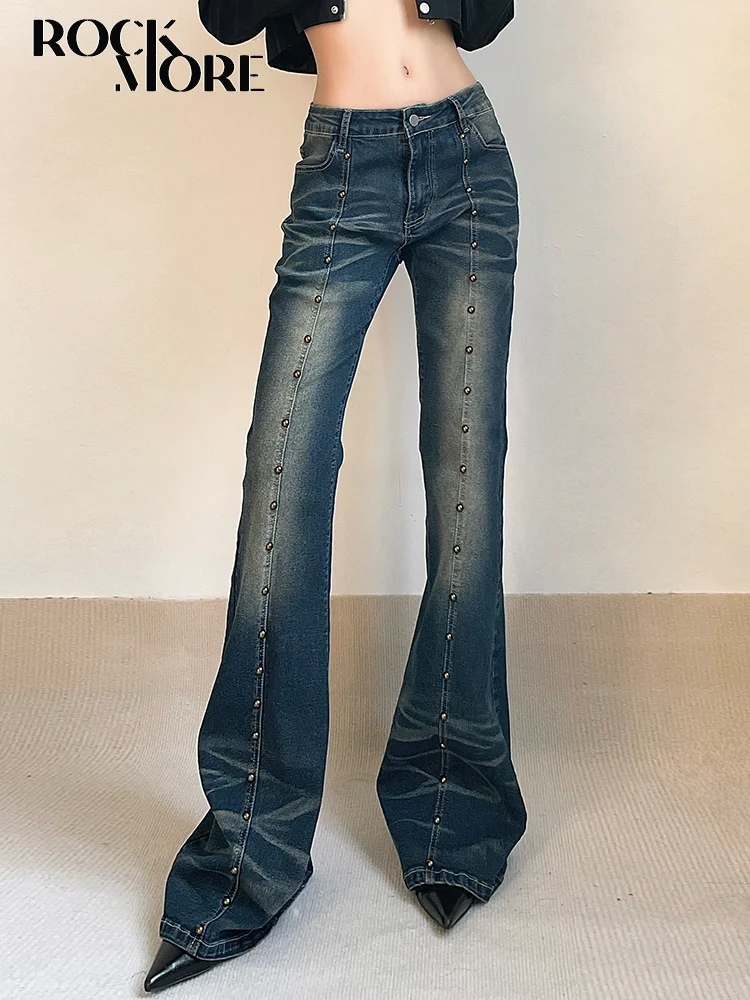This photograph, likely an advertisement for jeans, features a female model depicted from her mid-torso to her feet, with emphasis on the jeans. The model is wearing a very short black jacket that exposes her slender, bare stomach, and she has a small waist. The focal point of the image is the pair of dark denim jeans, which are designed with a slightly washed-out effect around the upper thigh, knee, and calf areas, giving them a rugged yet fashionable look. These jeans are exceptionally long, flaring out into bell-bottoms that completely cover her pointy black shoes, leaving only the tips visible. A distinctive line of nail-like buttons or rivets runs down the center of each leg from the waistband to the hem. The model stands on a beige carpet in front of a light tan, off-white colored wall. The word "Rockmore" is prominently displayed in black letters in the upper left corner of the image.